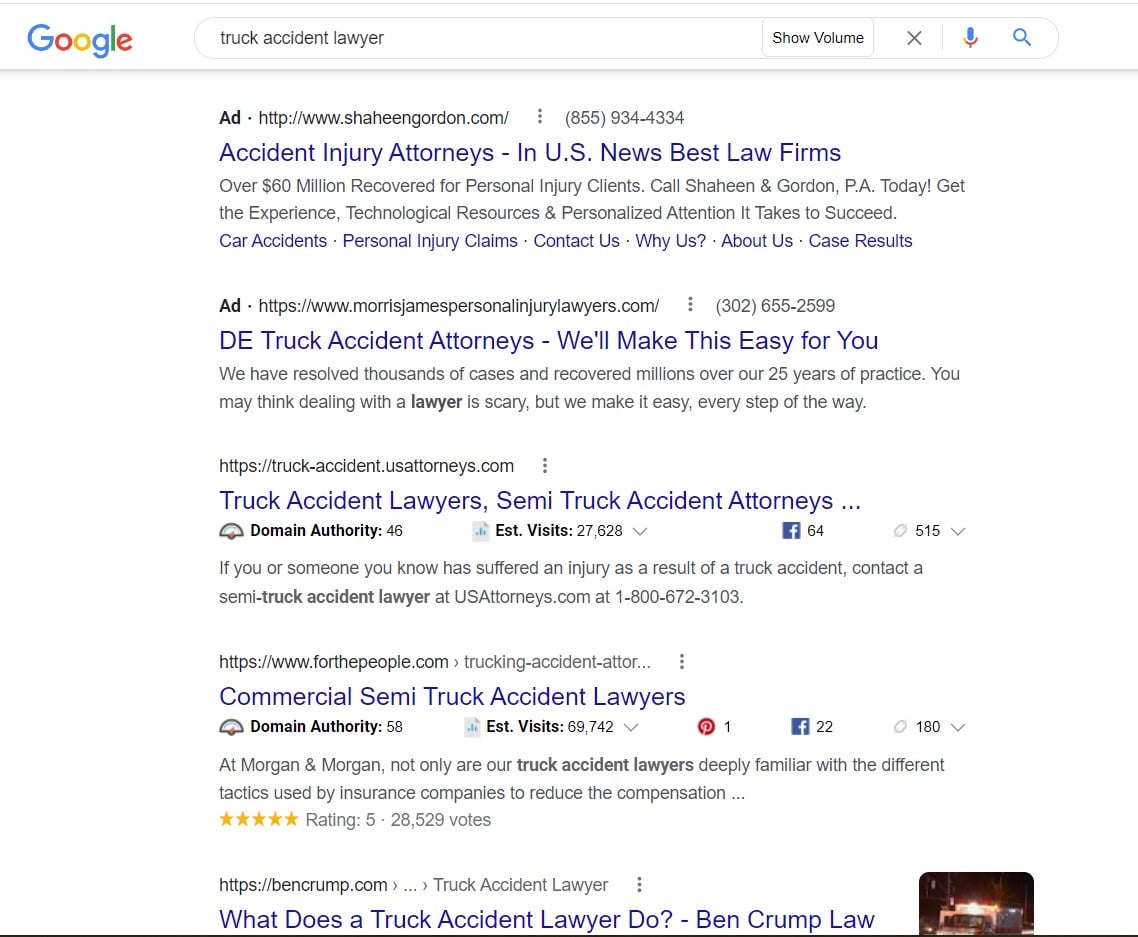This image captures the interface of a Google search results page. At the top, the iconic Google logo is prominently displayed with its distinct colors: a blue "G," a red "O," a yellow "O," a blue "G," a green "L," and a red "E." Below the logo, the search query entered is "truck accident lawyer."

The search results are led by sponsored advertisements. The first ad is from Shaheen & Gordon, P.A., promoting their services as accident injury attorneys across the United States, under the URL ShaheenGordon.com. The second ad also highlights personal injury lawyers and is hosted at MorrisJamesPersonalInjuryLawyers.com. The third result is an organic, non-sponsored link to truckaccident.usattorneys.com, which provides a directory of truck accident lawyers. The fourth result features Morgan & Morgan, a well-known firm advertised through their commercial slogan "For The People," which can be accessed at www.forthepeople.com. The final result presents Ben Crump’s legal services, accessible via BenCrump.com.

The layout is typical of a Google search results page, blending paid advertisements and organic search results, aimed at helping users find the legal assistance they need for truck accident cases.